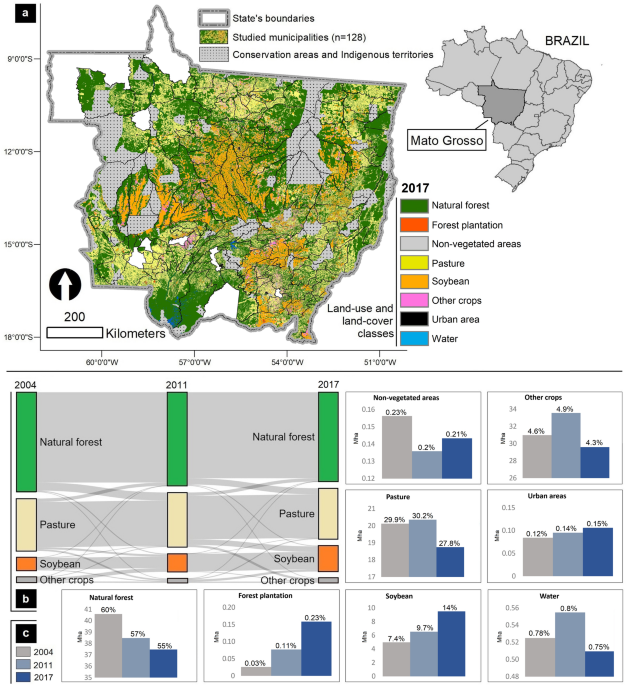This detailed image is a scientific map depicting the distribution of various land cover types within the state of Mato Grosso, Brazil, as of 2017. In the upper right corner, a gray outline of Brazil highlights Mato Grosso in dark gray. The main map to the left presents a color-coded visualization of land use within the state: dark green for natural forest, red for forest plantation, gray for non-vegetated areas, chartreuse for pasture, orange for soybean, pink for other crops, black for urban areas, and blue for water. The map includes coordinates on the X and Y axes, providing a precise overlay.

Beneath the map, multiple sets of bar graphs illustrate land cover changes over the years 2004, 2011, and 2017. These graphs break down the extent of natural forests, forest plantations, pastures, soybeans, other crops, non-vegetated areas, urban areas, and water bodies. The use of different colors—such as blue, gray, baby blue, green, tan, and orange—helps differentiate between these various categories. A scale at the bottom of the map indicates a distance of 200 kilometers. Overall, the image is highly detailed and scientific, providing a comprehensive overview of the land cover dynamics in Mato Grosso, Brazil.